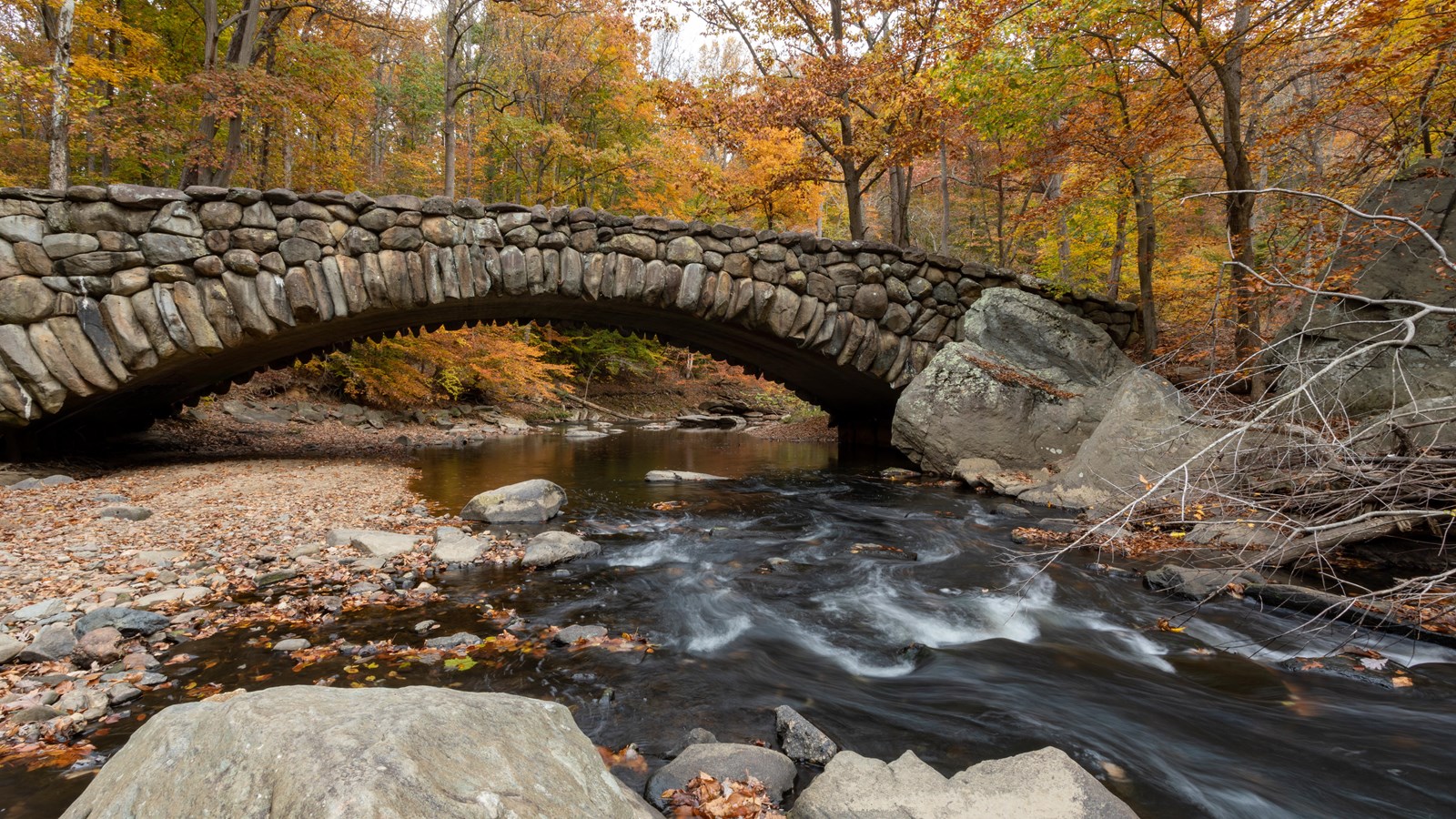This beautiful image captures an arched stone bridge spanning over a meandering creek amidst an enchanting autumn landscape. The creek, which appears to be rushing with turbulent water, is dotted with rocks, boulders, and scattered leaves. Some branches jut out from the water, adding to the natural complexity of the scene. Overcast skies cast a diffused light, enhancing the autumnal hues of green, brown, yellow, and orange in the surrounding trees. Tall rocks and numerous pebbles line the shore, giving texture to the serene yet dynamic setting. The bridge, constructed from large stones, gracefully arches over the clear water that flows from the right side of the image to the center, alluding to recent flooding in the mountainous areas upstream. The harmonious blend of natural elements and the tranquil, scenic backdrop captures the essence of a seasonal transition, portraying both calm and subtle movement in a long exposure photograph.